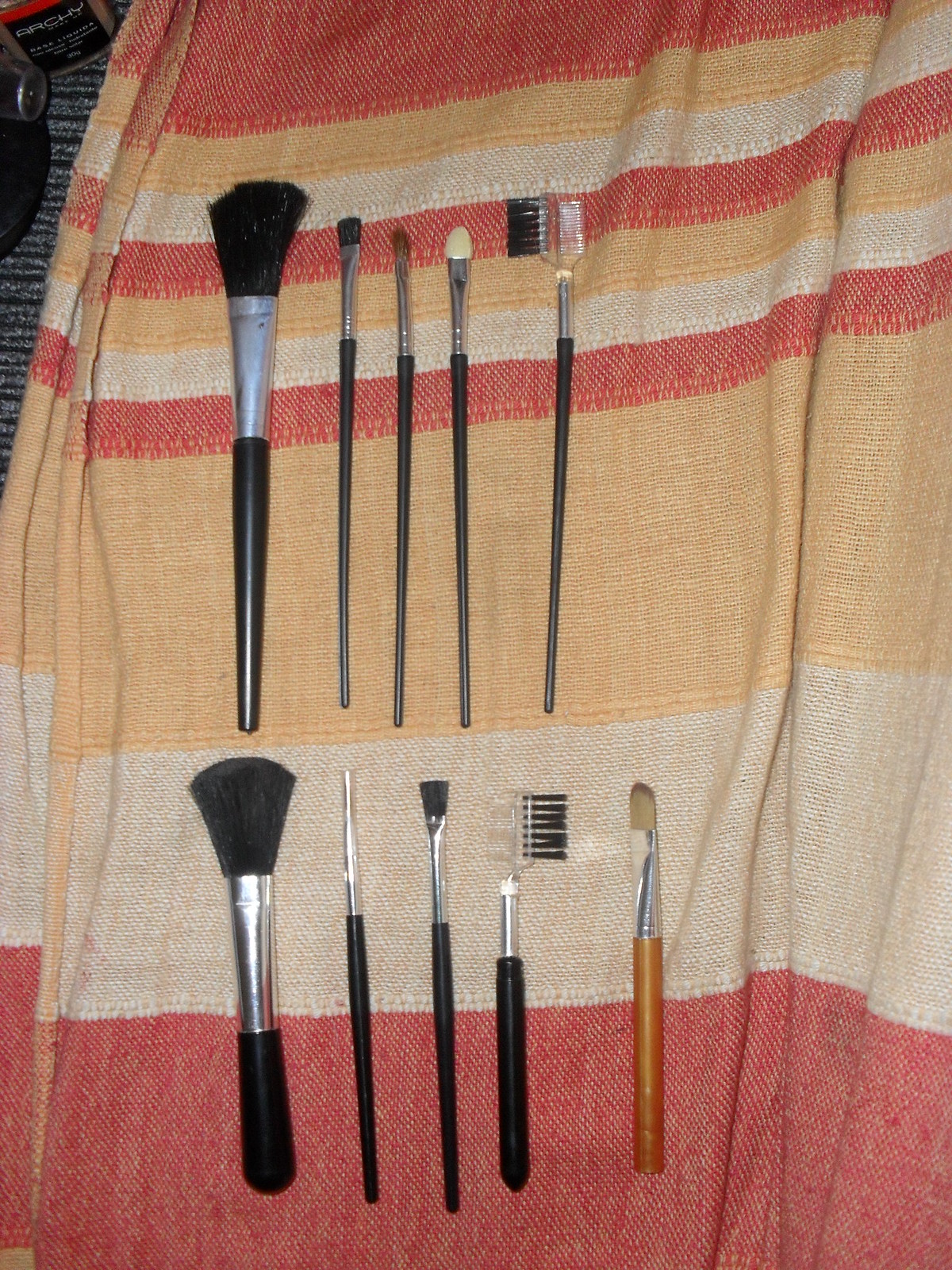The photograph showcases a meticulously arranged lineup of ten cosmetic brushes placed on a striped towel. The towel serves as a vibrant backdrop with its horizontal stripes in shades of red, yellow, and beige. The brushes are organized into two rows, each containing five items. Most brushes feature sleek black plastic handles with shiny silver metallic finials, except for one distinct brush with an orange-colored wood grain handle and a matching silver finial.

The top row features a variety of brush types: the first is a large, fluffy brush suitable for applying blush or powder, followed by two smaller brushes that resemble paintbrushes, likely intended for precise application. The fourth item is an eyeshadow applicator with a sponge tip, and the fifth is a versatile eyebrow comb/brush with dual ends — one for combing and the other for brushing.

In the bottom row, the first item mirrors the top row’s large, fluffy blush brush. The second item intriguingly lacks a brush head entirely. Following it are another paintbrush-like tool and then an eyebrow brush/comb featuring a left-positioned comb and an opposite brush. The sequence concludes with a final brush that also resembles a paintbrush in shape and functionality. The organized arrangement and careful detailing suggest that the brushes might have just been cleaned and are set out to dry on what appears to be a kitchen towel.